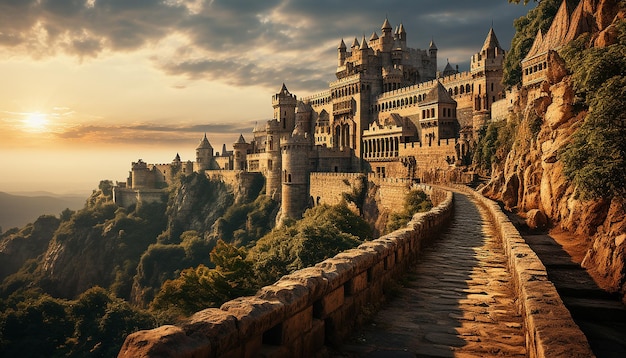The image depicts a stunning, possibly computer-generated scene reminiscent of an enchanting castle akin to Hogwarts. The castle, a massive and ancient structure constructed from gray concrete bricks, stands majestically on the side of a mountain. Its grandiosity is highlighted by numerous windows and various pointed roofs adorned with circular watchtowers. To reach this architectural marvel, a long cobblestone pathway winds through the center of the image, flanked by ledges that open to an array of treetops, bushes, and grassy cliffs. The left corner of the image captures a mesmerizing sunset, casting a warm yellow glow that enhances the tan-gray hue of the castle and illuminates the light gray sky dotted with dark clouds. This ethereal scene is further accentuated by the rocky hill on the right side, topped with patches of grass and trees, completing the picturesque landscape. The setting is both grand and serene, with the castle towering imposingly yet harmoniously within its natural surroundings.